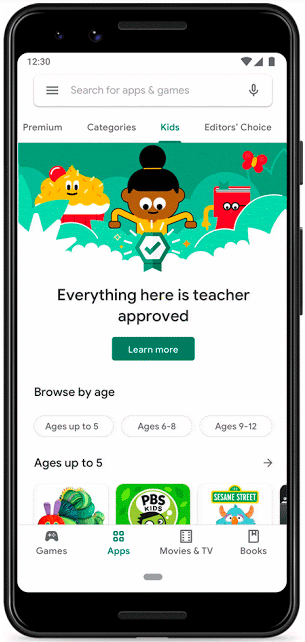The image is a detailed screenshot of a phone screen displaying an app or web page, resembling a hand-drawn picture. The phone's black case and top edge are visible. At the top of the screen, the time reads 12:30. A search bar labeled "Search for apps and games" is prominently displayed beneath the time.

Below the search bar, there are several categories listed: "Premium," "Categories," "Kids," and "Editor's Choice." Featured prominently is a colorful cartoon illustration. The illustration includes a yellow, white, and red sundae topped with a cherry, a black child with black hair wearing a yellow shirt, a sentient red book with eyes and hands, a red butterfly, and a check mark beneath the girl. The text accompanying this image reads, "Everything here is teacher approved," followed by a green rectangular button labeled "Learn More."

Further down, the section labeled "Browse by Age" categorizes content into age groups: "Ages up to 5," "Ages 6 to 8," and "Ages 9 to 12." Under the "Ages up to 5" section, an arrow points to the right, leading to three squares titled "Games," "PBS Kids," and "Sesame Street," each featuring a corresponding image above the text. Additional buttons for "Apps," "Movies and TV," and "Books" are listed below these squares.